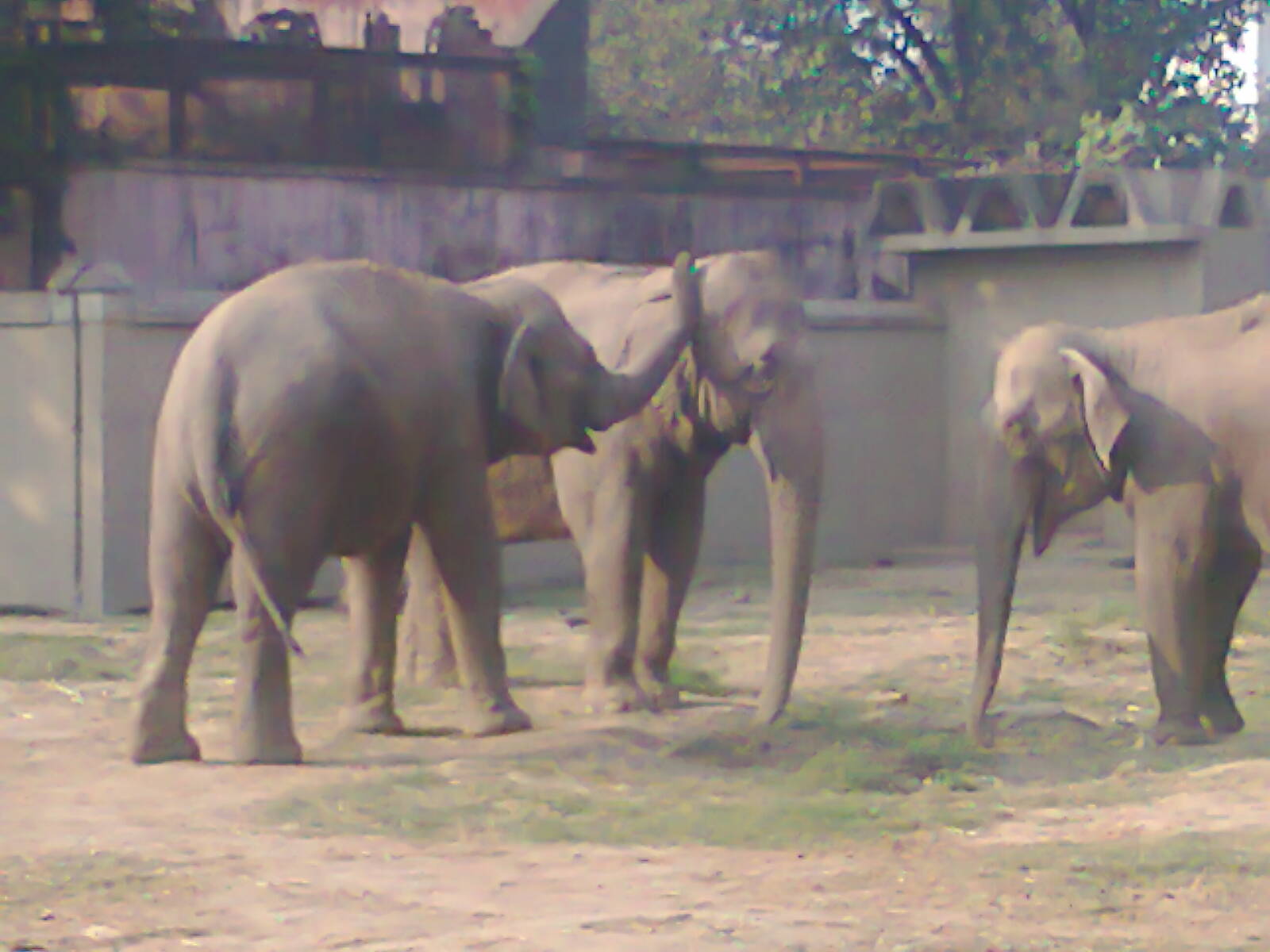This photograph depicts three large, gray Indian elephants in a zoo enclosure. The image is slightly blurred and lacks sharpness and contrast, but the details remain discernible. The elephants are situated on a tan dirt floor interspersed with sparse patches of short grass. They appear to be in a huddle: the elephant on the left is seen resting its trunk on the head of the elephant in the center, whose trunk is touching the ground. The third elephant, partially visible on the right, also has its trunk resting on the ground and appears to be approaching the other two. The enclosure is delineated by a tall, gray concrete wall, which is partly topped by a taller, white wall and some brown construction elements, possibly part of the zoo’s infrastructure. In the background, a large leafy green tree is visible in the top right corner, adding a touch of foliage to the otherwise structured environment. The composition of the photograph, despite its softness, captures a candid moment of interaction among the elephants in their captivity.